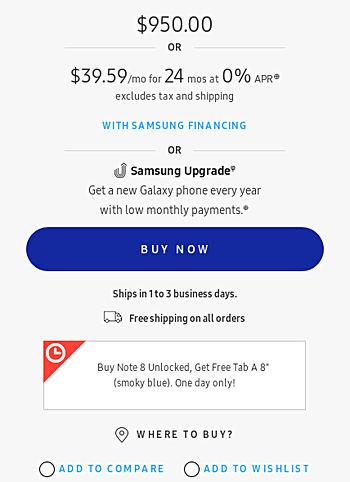Discover unbeatable deals with Samsung’s latest Galaxy phone offer. For only $950 upfront or $39.59 a month for 24 months with zero interest through Samsung Financing or the Samsung Upgrade Program, you can unlock a world of possibilities. Please note that taxes and shipping are extra. Enjoy the convenience of getting a brand-new Galaxy phone every year with affordable monthly payments.

A large blue "Buy Now" button prominently invites you to take advantage of this offer, ensuring your new device ships within one to three business days with free shipping on all orders.

Additionally, seize the exclusive one-day offer of a free Tab A8 in Smoky Blue when purchasing an unlocked phone. For further convenience, a "Where to Buy" section lets you find various purchasing locations nearby.

At the bottom of the page, you'll find two handy buttons: "Add to Compare" and "Add to Wish List," helping you make the best decision and keep track of your favorite products.

This promotion is your gateway to the latest Samsung technology with unmatched financing flexibility and additional perks.